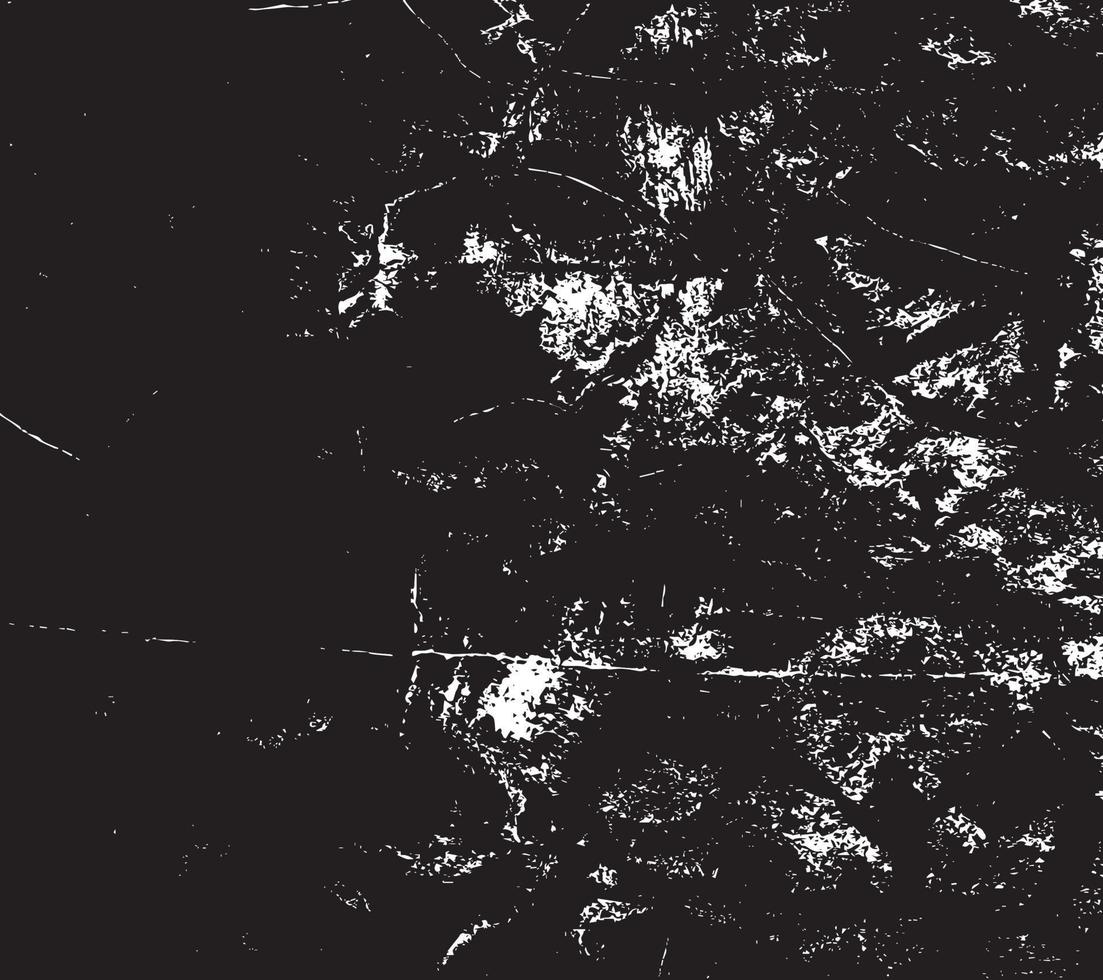The image resembles an artistic blotched black background with numerous irregular white splotches, creating an abstract, almost Rorschach-like appearance. Predominantly concentrated on the right side, these splotches and various white lines contrast starkly against the deep black, evoking an impression of hidden faces or mysterious figures. A prominent white line runs horizontally across the center, adding to its enigmatic quality. The left side is more subdued with fewer markings, while the overall aesthetic might evoke interpretations ranging from space and starry skies to looking upward through a canopy of trees. It embodies a minimalist, monochromatic style that could incite varying reactions, encapsulating the essence of modern abstract art you'd encounter in a museum.